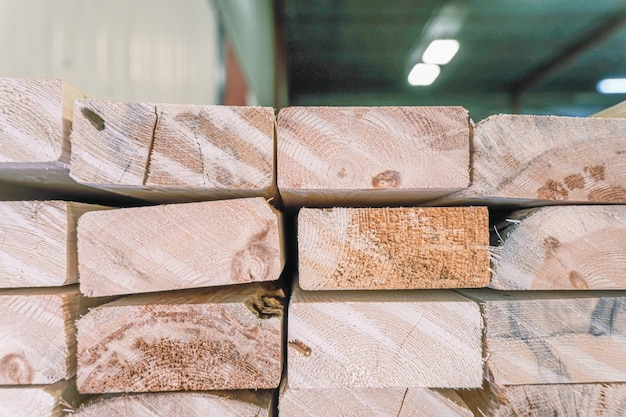This image features a close-up photograph of neatly stacked lumber, specifically 2x4 wood blocks, arranged in at least four rows and four blocks high. The blocks are cut into perfect rectangular shapes, exhibiting a mix of quarter-sawn and plain-sawn cuts, revealing distinctive growth lines and varied grain patterns. Some blocks display natural knots, and the color of the wood ranges from light beige to golden hues. The end grains of 16 blocks are prominently visible, showcasing the varied shades and textures of the wood. The photograph captures the scene indoors, with a blurred background that appears to be a warehouse or facility. The ceiling is a dark green metal structure featuring two small rectangular lights in the center and a small white rectangular light on the right-hand side, all turned on and illuminating the scene. Additionally, there is some natural light present, complementing the artificial illumination. The wood blocks take up the bottom two-thirds of the image, framed against the softly focused backdrop.